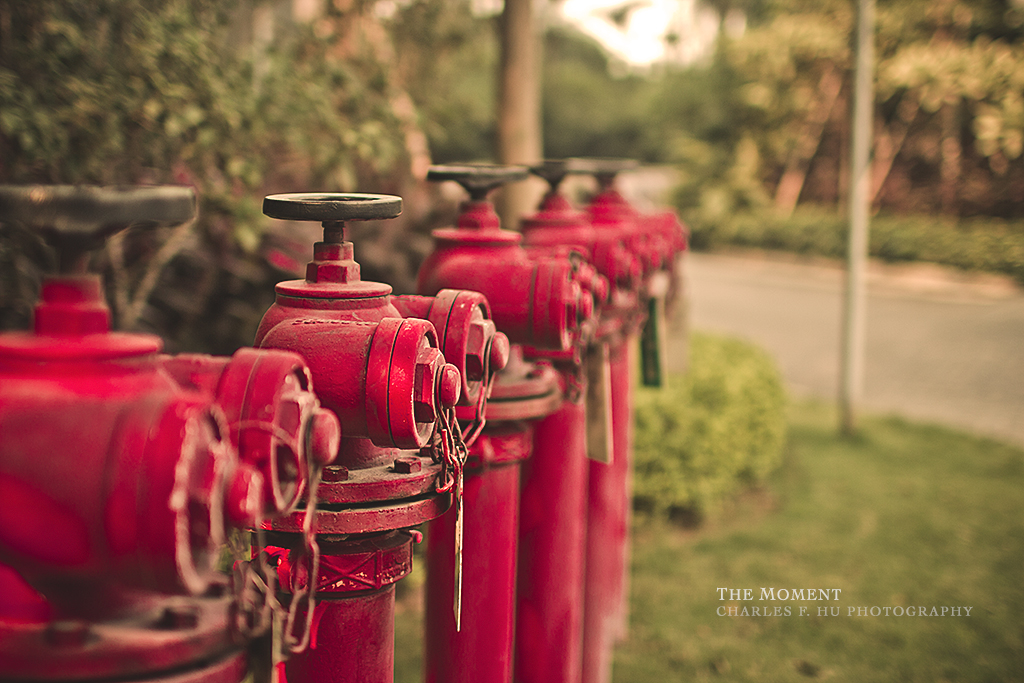This detailed photograph captures six red fire hydrants lined up in a row, their streamlined design emphasizing slender, upright pipes bolted together. Each hydrant features a black, metallic control valve at the top and has chains linking to two hexagonal bolts. The hydrants in the foreground are sharp and clear, while those in the background progressively blur. Behind them, a lush backdrop of green trees, bushes, and grass is evident, with a road cutting across the scene and more trees on the other side. A pole is visible near the street, contributing to the urban context. At the bottom right corner of the image, a white watermark reads "The Moment. Charles F.H.U Photography," indicating the photographer’s signature.